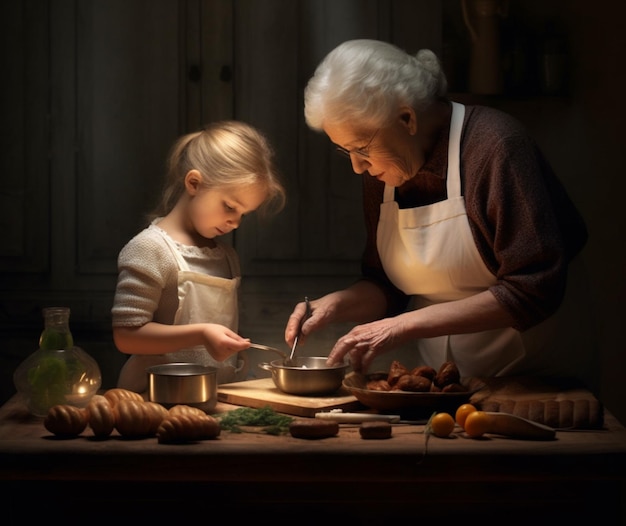The image depicts a detailed and realistic scene, possibly computer-generated, of a grandmother and a young girl cooking together under a single, overhead light source that casts a dramatic illumination on their activity. The background is all dark, focusing the viewer's attention on the pair and the table of ingredients before them. The table, wooden and centrally positioned, holds a cutting board with a silver bowl or pot into which both the grandmother, on the right, and the young girl, on the left, are placing ingredients with their respective spoons. The grandmother, with coiffed gray (or white) hair and glasses, is dressed in a brown top and white apron, while the girl has blonde hair pulled back into a ponytail and wears a white-gray top with a white apron. The table is scattered with various ingredients, including a glass jar with liquid, several bread rolls or croissants, green herbs, orange carrots, some green vegetables, and an assortment of unidentified fruits or vegetables. The overall mood is intimate and focused, showcasing the shared activity in the warmth of their collaboration.